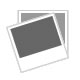This is an old sepia-toned black-and-white photograph, approximately three and a half inches wide, as indicated by the green ruler marked "Made in USA" at the bottom of the image. The woman in the photograph appears to be Japanese, likely in her early to mid-twenties, and is seated against a plain gray background. She is dressed in a traditional Japanese kimono adorned with a floral or circular stem pattern and a wide obi sash around her waist. Her hair is styled up, possibly held with a clip, and she has a serene expression, gazing slightly off-camera to the left without smiling. The photograph has notable damage, with visible spots of degradation particularly in the top left and bottom left corners, likely from handling. The image has a black border lined with a thin white line. At the bottom right corner of the photograph, there is an embossed name, "Akamatsu," followed by some unreadable text that also appears to be in Japanese. The overall quality of the photograph is poor, with noticeable fading around the woman.